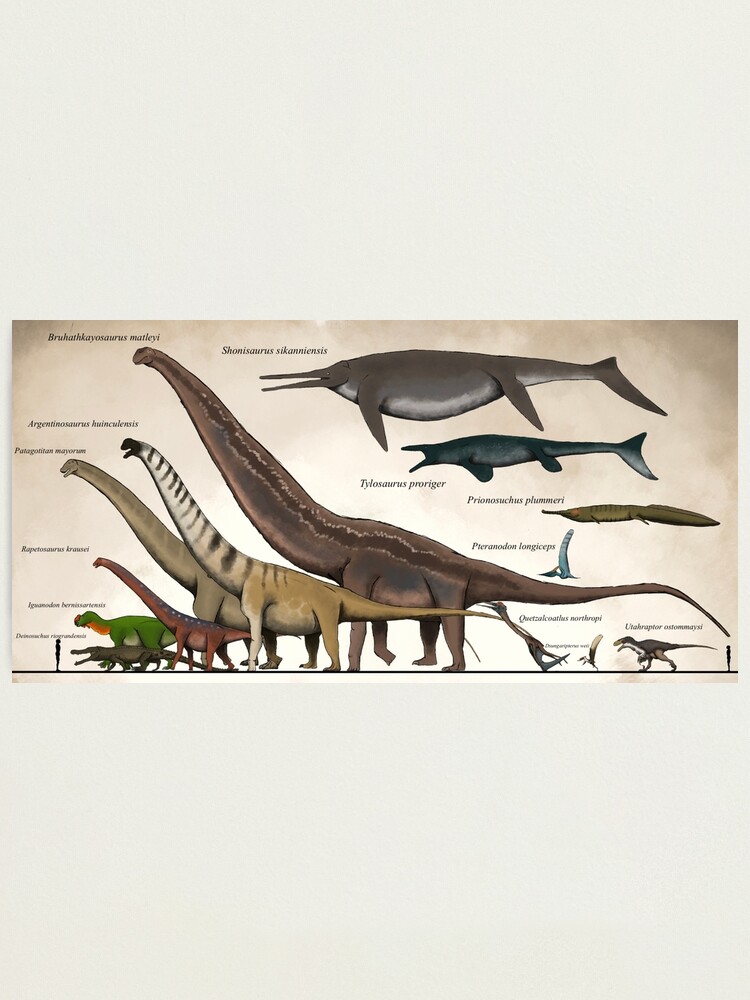This image, in portrait layout, is divided into three equal horizontal segments. The top and bottom thirds feature a solid off-white, cream color. The middle third, which also has a cream-colored background, showcases an array of various dinosaur illustrations. 

On the left side of the middle segment, there is a small human figure for scale comparison. Next to the human is a creature resembling an alligator, followed by a series of dinosaurs of varying sizes and colors. The dinosaurs include one that is green, another that is reddish, a brown one, a black and tan striped one, and another brown dinosaur. 

Behind this row of dinosaurs are two smaller dinosaurs: one appears to have wings, reminiscent of a pterosaur, and the other resembles a small, brown T-rex. In the upper right-hand corner of the middle segment, four different kinds of fish are depicted, seemingly floating. Each animal, whether dinosaur, human, or fish, has its corresponding genus and species labeled next to it in text.